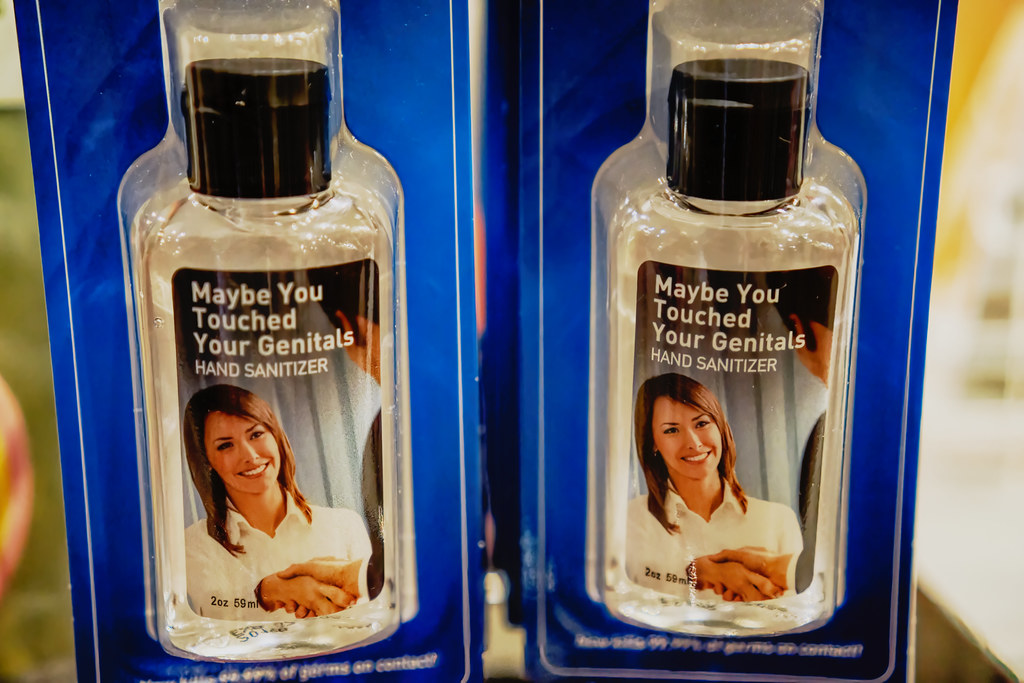This image showcases two identical packages of gag gift hand sanitizers, displayed in rectangular blue packages with white pinstripes. Each package contains a tiny, 2-ounce (59 milliliters) clear liquid hand sanitizer in a transparent plastic casing, revealing a black flip cap bottle. The front label of the bottle humorously reads, "Maybe You Touched Your Genitals Hand Sanitizer," in white text. The label also features an image of a smiling Caucasian woman shaking hands with a man, of whom only the back left side of his head is visible. The background of the photo is blurred, with hints of greens, yellows, and other colors, adding focus to the comically captioned hand sanitizers in the foreground.